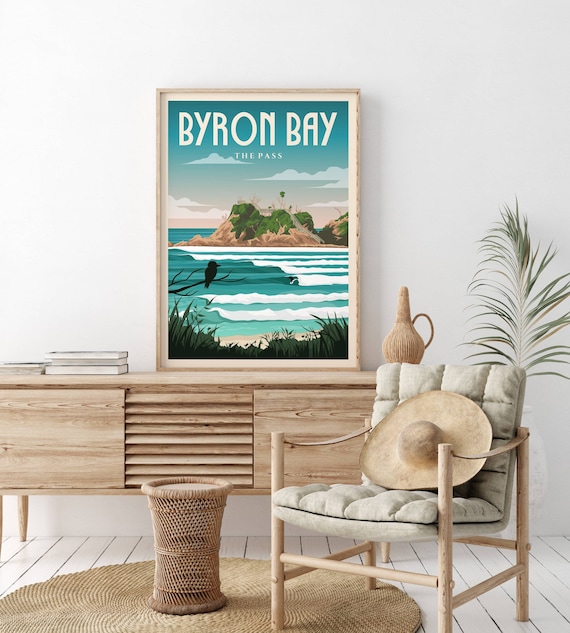This vertical rectangular image depicts a meticulously curated coastal-themed living room with a fresh, beachy atmosphere. The background features pristine white walls and a white wood plank floor. Central to the image is a light tan wicker circular rug, upon which stands a cylindrical wicker side table. Adjacent to the table is a rustic light brown wooden chair with a light green cushion, adorned with a large tan sun hat. Behind this, against the crisp white wall, is a light wood entertainment console featuring two side doors and horizontally slatted shelves in the center. The console holds a few books to the left and a wicker pot to the right. Leaning against the wall atop the console is a framed artwork showcasing a serene beach and ocean scene, complete with a volcanic mountain and tall grasses, with the inscription "Byron Bay, the pass." Flanking the composition is a tall plant, adding a touch of natural greenery to the scene. The overall arrangement evokes a tranquil, beachside retreat, perfect for relaxation and leisure.